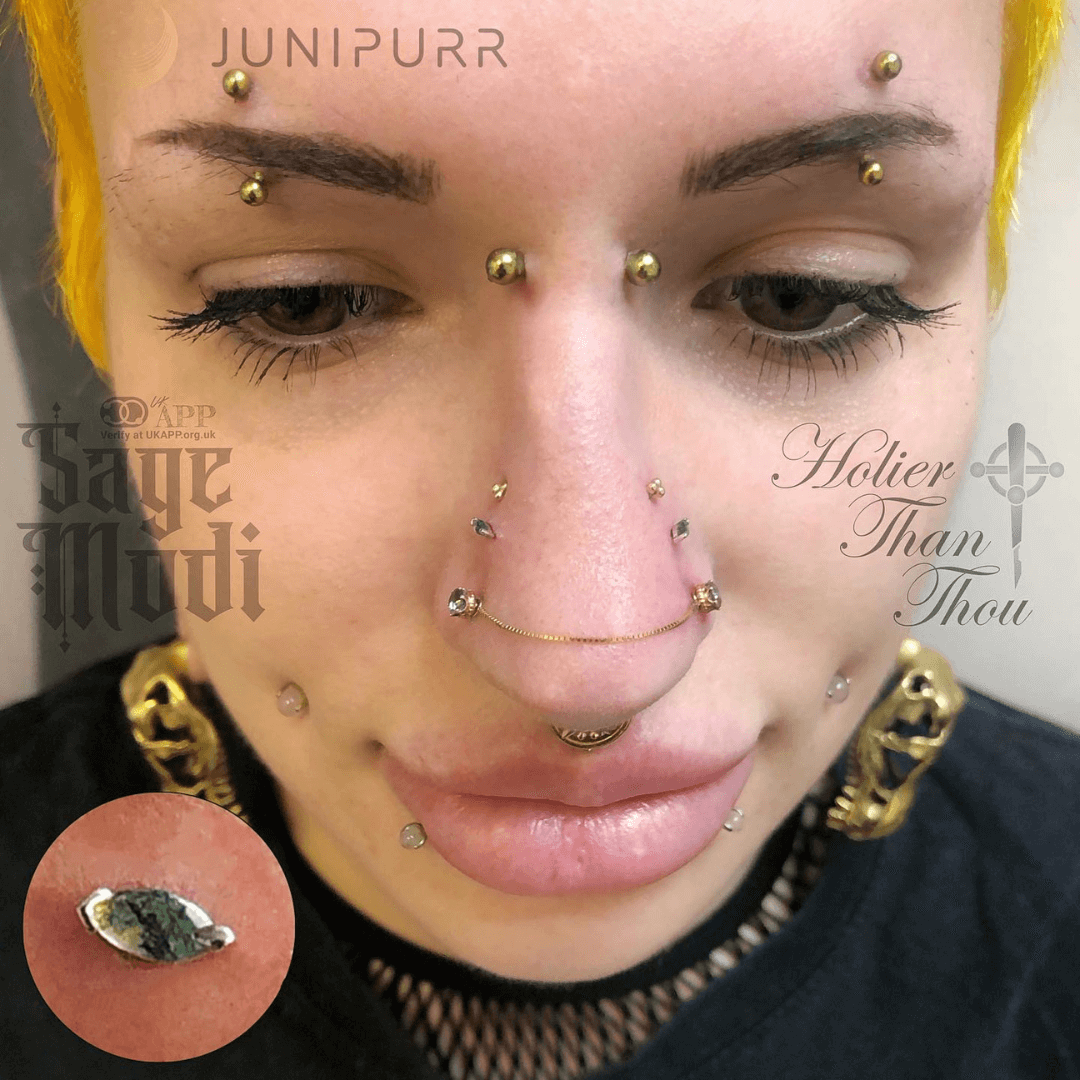The image is a close-up of a Caucasian woman with an extensive array of facial piercings and a distinctive appearance. She has platinum yellow hair and large pink lips. Her eyebrows each have a piercing above and below them. She sports three piercings on each side of her nose, with the bottom ones connected by a small chain, and a septum piercing hanging from the center of her nose. Additionally, her nose bridge is adorned with a series of piercings that stretch from the nostrils up towards the eyes. Her cheeks are pierced with small pearls, and she has two piercings on either side of her bottom lip featuring small glass bulbs. There are piercings on her eyelids, made from golden bulbs. She is wearing a black shirt and multiple pieces of golden jewelry, including a noticeable golden necklace. There is text overlaid on the image: "Junipur" in the top left, "Sage Modi" in the middle left, and "Holier Than Thou" with a scalpel and barbell cross on the right side.